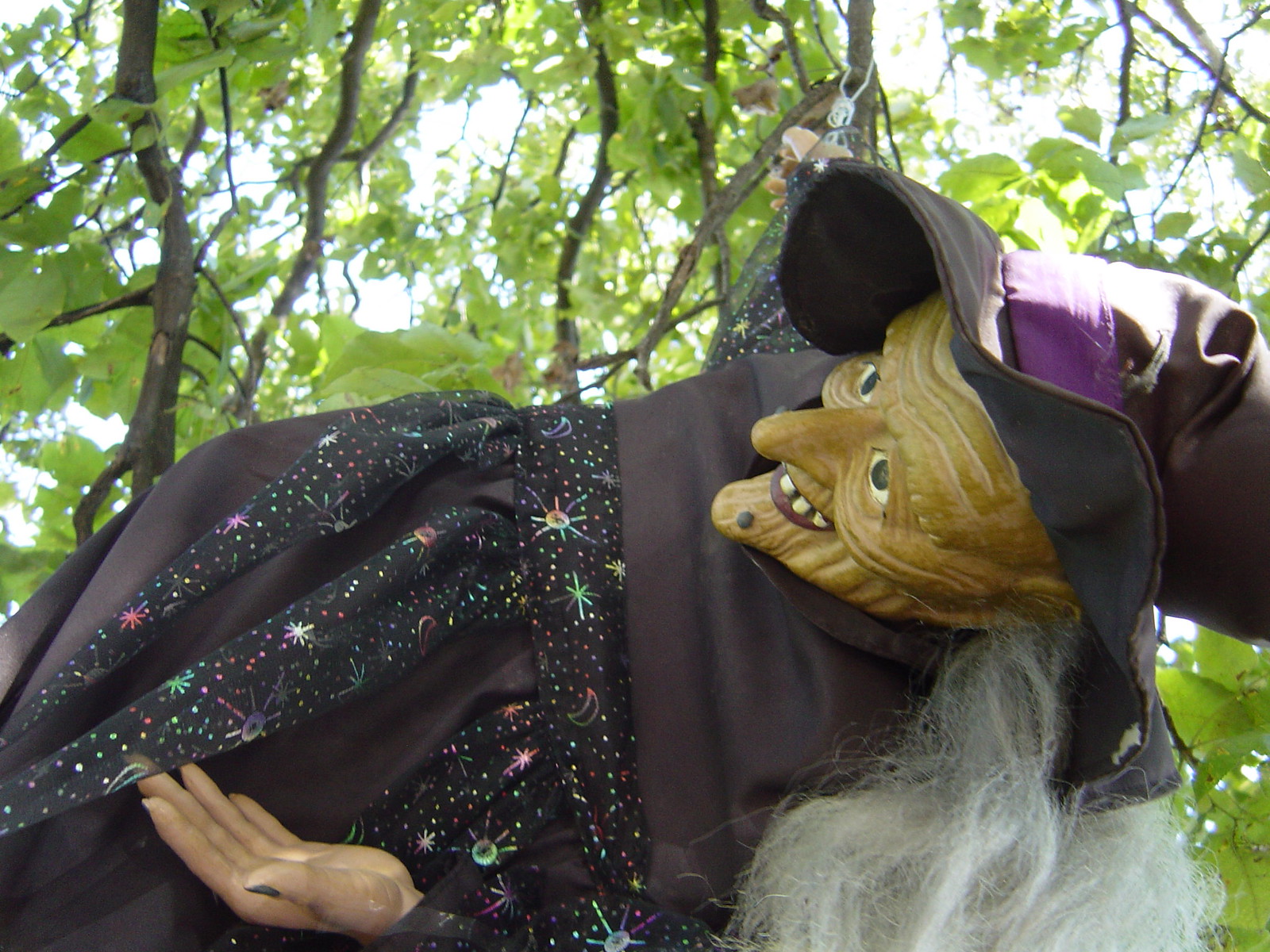The image depicts a Halloween decoration of a witch figure, appearing like a mannequin made of rubber. The witch has an eerie, olive green face with scraggly, white hair peeking out from under a black hat adorned with a purple stripe. Her facial features are exaggerated and grotesque, with a long, pointy nose, a prominent dark mole on her chin, ugly teeth, dark lipstick, and a plethora of wrinkles. She wears a black dress which is decorated with colorful piping, ribbons, stars, and other embellishments. The figure hangs sideways from a tree branch in a horizontal position, specifically dangling by her right arm, while her rubber left hand rests down near her side. The backdrop consists of tree leaves, brown branches, and glimpses of the sky, emphasizing the outdoor setting. The overall presentation hints at someone creatively using this decoration to add a spooky atmosphere to the scene.